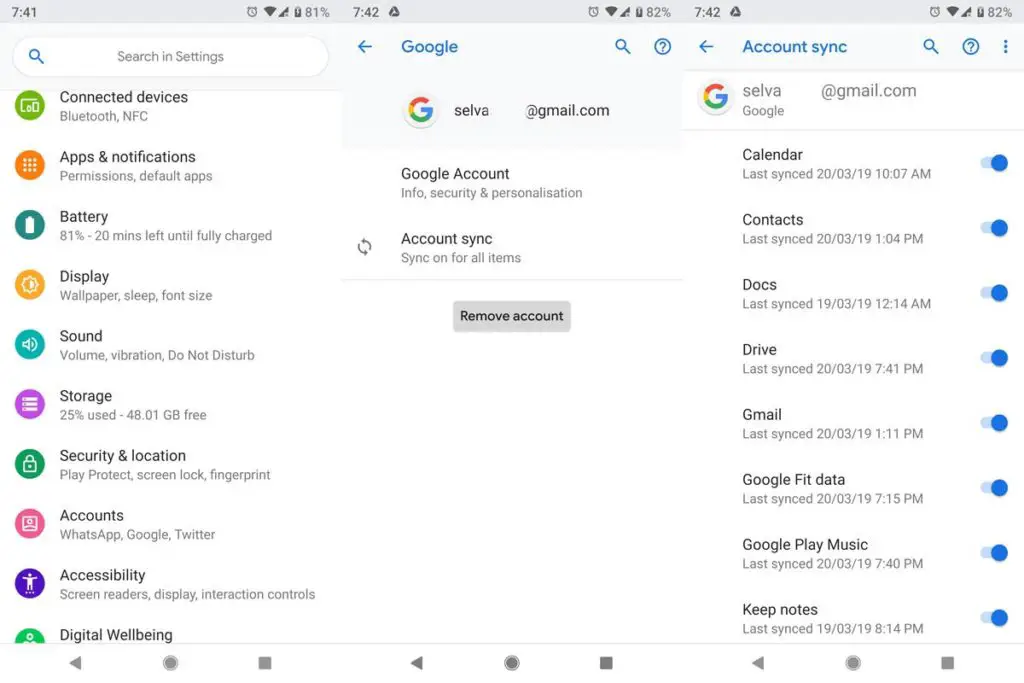The image depicts a detailed settings page with a predominantly light off-white background. At the top, there's a light gray rectangular bar displaying the times 7:41 and 7:42, interspersed with icons for an analog clock, Wi-Fi signal, and battery indicators showing levels of 81% and 82%. 

Below this, from left to right, is a lengthy white oval containing a blue magnifying glass icon on the left, accompanied by black text that reads "Search in Settings." Next to it is a blue left-pointing directional arrow, blue text stating "Google," followed by another blue magnifying glass, a circle with a question mark inside, another blue left-pointing arrow, blue text that reads "Account Sync," another blue magnifying glass, a circle with a question mark, and finally, three vertical blue dots.

Along the left-hand side, vertically aligned, are the following menu options: 
- "Connected Devices," with sub-options like Bluetooth and NFC.
- "Apps & Notifications," including permissions and default apps.
- "Battery," showing 81% with 20 minutes left until fully charged.
- "Display," covering wallpaper, sleep, and font size.
- "Sound," detailing volume, vibration, and Do Not Disturb settings.
- "Storage," indicating 25% used with 48.1 GB free.
- "Security & Location," featuring Play Protect, screen lock, and fingerprint.
- "Accounts," listing connected accounts like WhatsApp, Google, and Twitter.
- "Accessibility," describing screen readers, display adjustments, and interaction controls.
- "Digital Wellbeing."

In the center of the page, a Google emblem appears with the email address "selva@gmail.com." This section includes:
- "Google Account" information on security and personalization.
- "Account Sync," showing sync for all items and an option to remove the account.

On the right, associated with "selva@gmail.com," synchronization details are listed for various Google services:
- Calendar: Last synced on 23-19-10-07 AM.
- Contacts: Last synced on 20-03-19-10-04 PM.
- Docs: Last synced on 19-03-19-12-14 AM.
- Drive: Last synced on 20-03-19-7-41 PM.
- Gmail: Last synced on 20-03-19-11 PM.
- Google Fit Data: Last synced on 20-03-19-7-15 PM.
- Google Play Music: Last synced on 20-03-19-7-40 PM.
- Keep Notes: Last synced on 19-03-19-8-14 PM.